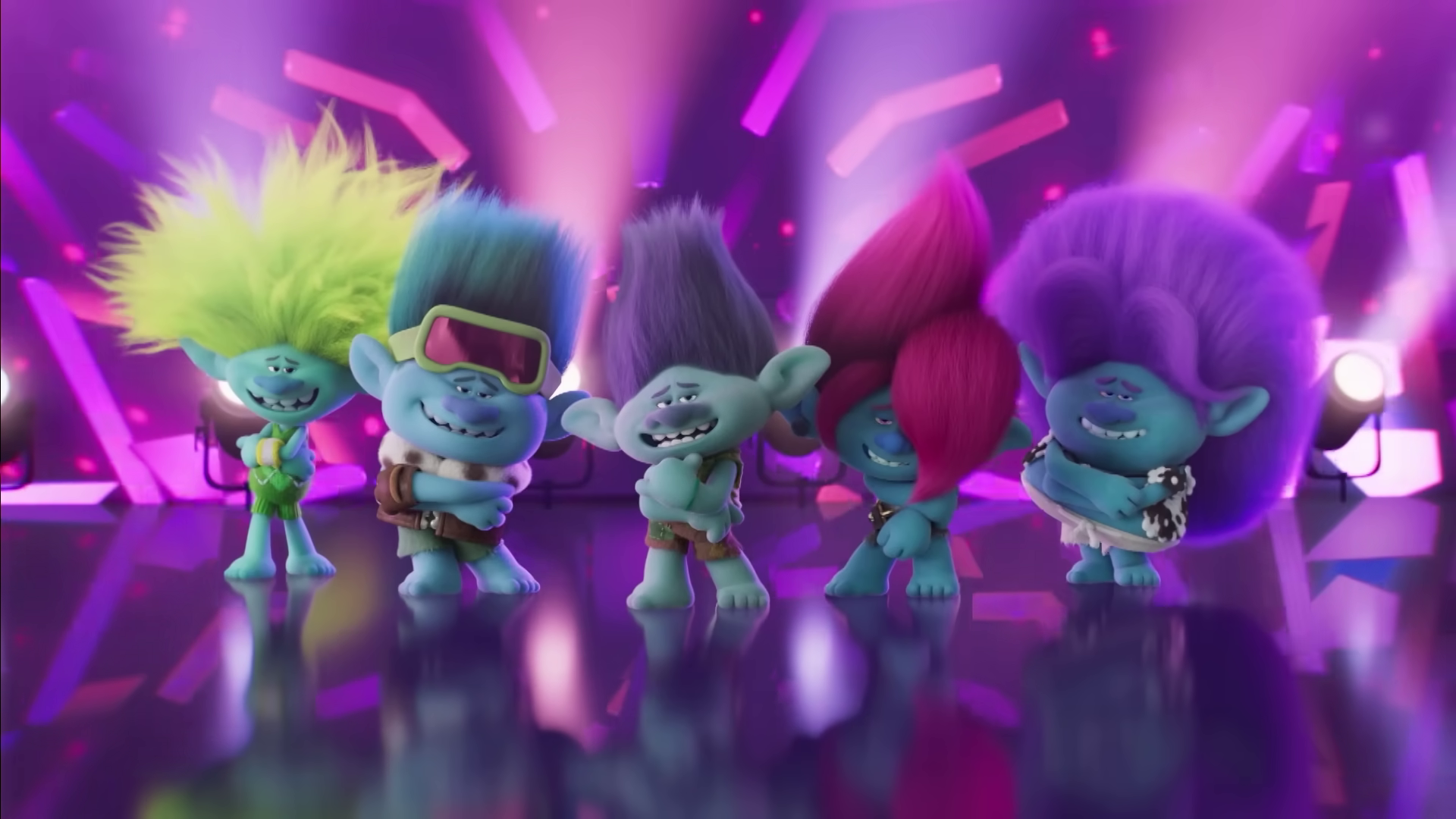This is an image of five colorful cartoon characters resembling Smurfs or trolls, each with unique characteristics and vibrant hairstyles. These small beings, primarily seafoam green or turquoise in color, stand on a glossy, reflective purple floor. The background is a vivid mix of purple and pink with a confetti-like effect comprising small dots and dashes, reminiscent of broken or bent straws scattered behind them. The character on the far left sports yellow hair and a matching yellow outfit, distinguishing him from his companions. Moving right, the next character has seafoam green hair sticking up with glasses on top, followed by one with upright purple hair. Another character has distinctive pink hair styled in a coiffed manner, with one piece going straight up and another draped over their left eye. The character on the far right features large, fluffy purple hair, with two pieces puffed up in the front and the remainder slicked back in a poof. This lively and dynamic scene is set against a background that is illuminated in shades of purple and pink, adding to the whimsical nature of the image.